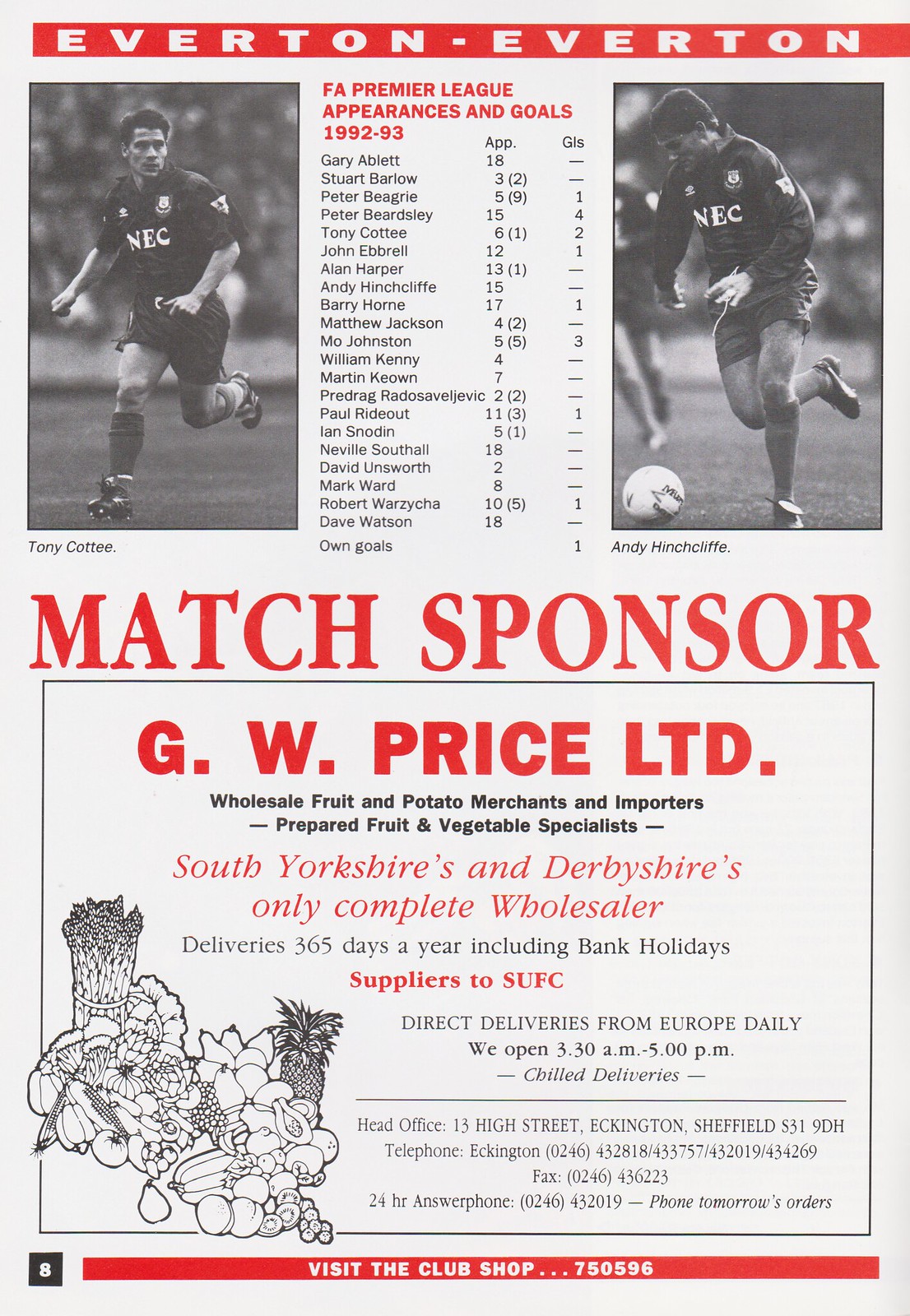This detailed poster advertises a soccer match in the FA Premier League from the 1992-1993 season. At the top, "Everton / Everton" appears in white text against a red background. Below, two black-and-white images feature soccer players flanking a central roster and scoreboard. The left side shows a player running with "NEC" on his jersey, while the right side depicts another player kicking a ball. Centralized red text reads, "FA Premier League appearances and goals 1992 to 1993," listing approximately 15-16 players and their achievements.

Beneath the player statistics, the match sponsor is prominently highlighted in big red letters, reading "Match Sponsor." A black-bordered box contains further details about the sponsor: "G.W. Price Ltd. - Wholesale Fruit and Potato Merchant and Importers, Prepared Fruit and Vegetable Specialists." This text is black on a white background. Additional information specifies that G.W. Price operates in South Yorkshire and Derby Shires, delivering 365 days a year, including bank holidays, and supplying SUFC. Drawn sketches of various fruits and vegetables, including pineapples, asparagus, lettuce, pears, and watermelon, appear just below this text. A smaller black print to the right mentions, "Direct deliveries from Europe daily."

Finally, a red horizontal bar at the bottom urges viewers to "visit the club shop" in white print. The flyer itself employs a color scheme dominated by red, white, and black, giving it a distinctly aged appearance reflective of its early 1990s origin.